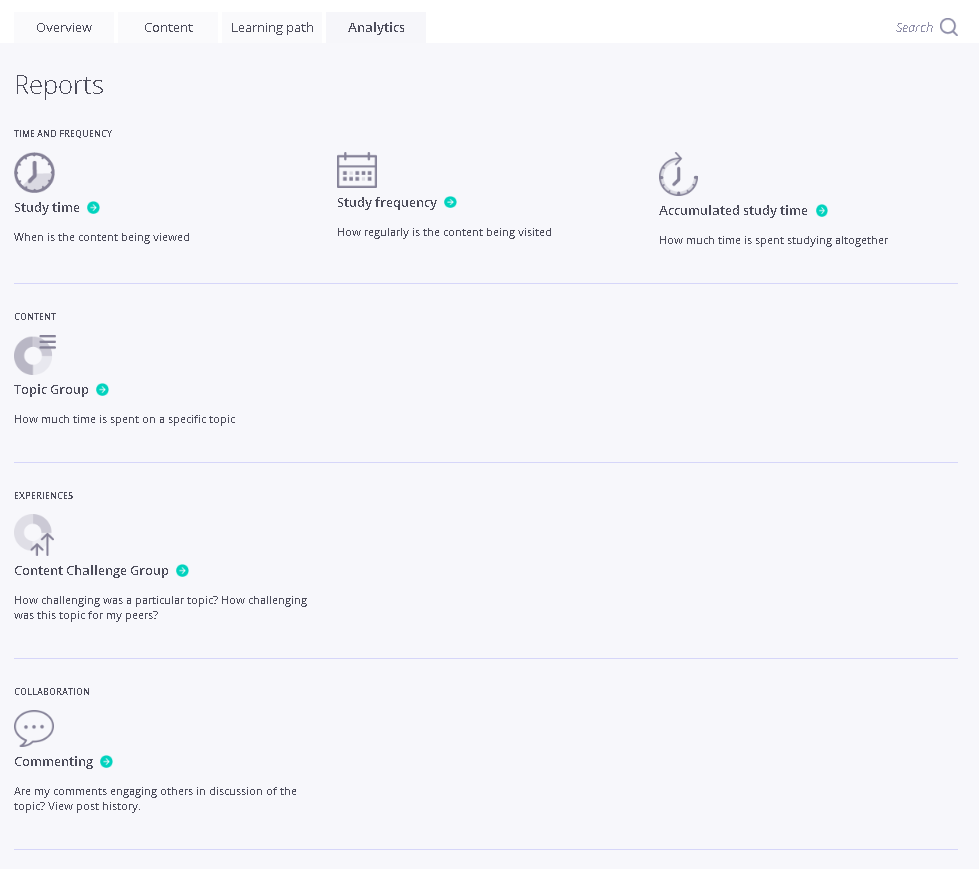Screenshot of a detailed analytics report page from a study platform, rendered against a grayish-colored background. The interface is organized with potential tab options such as "Overview," "Content," "Learning Path," and "Analytics," with "Analytics" being the currently active tab. 

### Upper Section:
- **Search Bar**: Located in the upper right-hand corner, featuring a white background with a search icon, contrasting with the overall gray backdrop of the page.

### Main Analytics Section:
- **Reports Description**: Below the "Analytics" tab, the page is titled "Reports," focusing on "Time and Frequency."
  - **Study Time Section**:
    - **Clock Icon**: Accompanies the label "Study Time," which explains when the content is being viewed.
    - **Calendar Icon**: Paired with "Study Frequency," detailing how often the content is accessed.
    - **Accumulated Study Time**: Represented by a half-clock with an arrow icon, indicating the total amount of time spent studying.

### Mid-Section:
- **Gray Divider Lines**: Subtle gray lines separate different sections of content for clear delineation.
  - **Content Topic Group**: Specifies the amount of time spent on particular topics.

### Lower Section:
- **Experiences Section**:
  - **Content Challenge Group**: Evaluates how challenging specific topics are for both the user and their peers.
  - **Collaboration Section**: Marked by a message icon, focusing on engagement metrics such as commenting and the effectiveness of comments in fostering discussions, also featuring a "View Post History" option for further details.

This well-structured and descriptive analytics report page offers in-depth insights into study habits, content engagement, and peer comparisons.